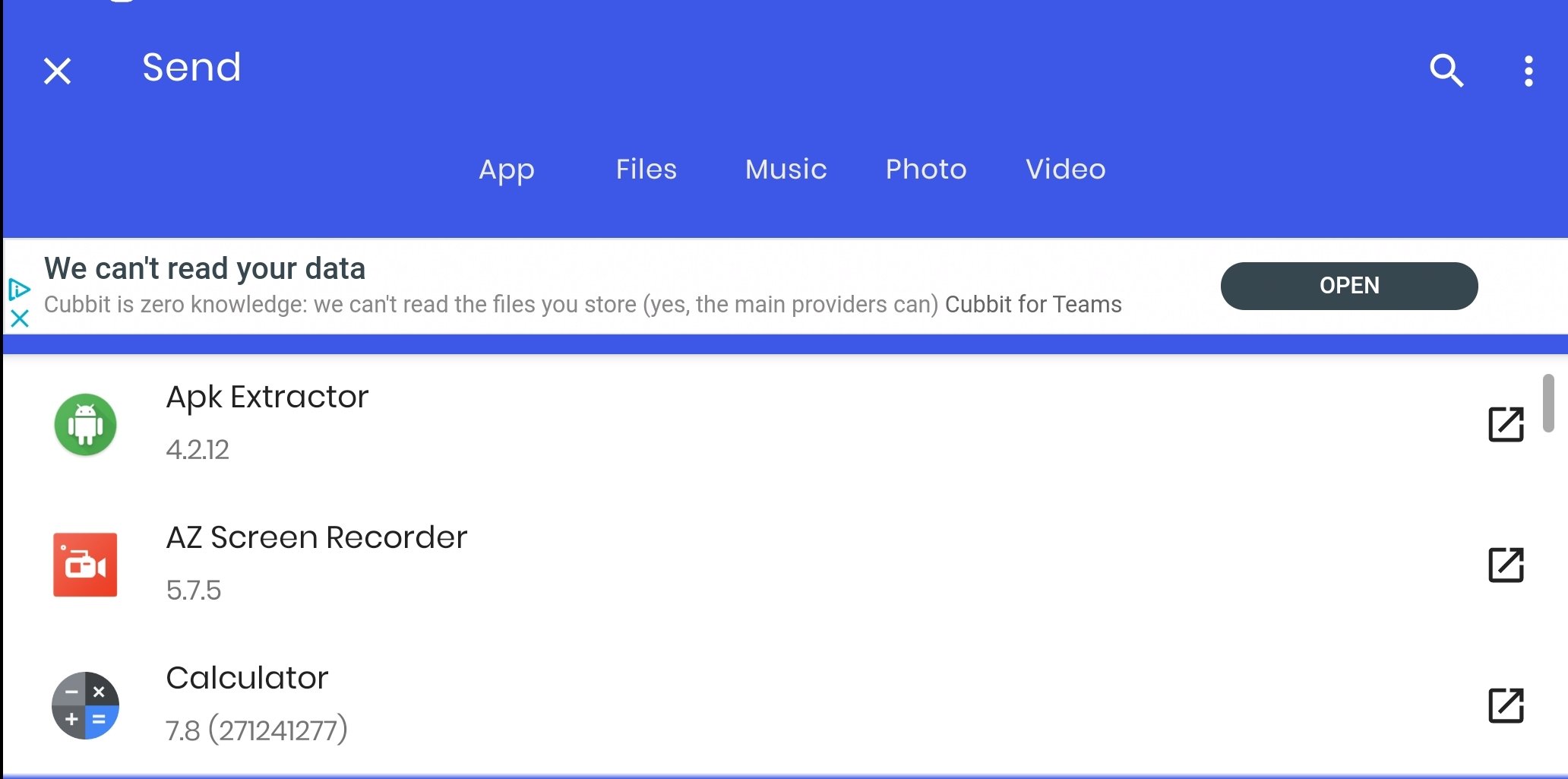The interface depicted appears to be a settings menu for a device or an application. The header is adorned with a purple-blue gradient and white text, featuring various interactive elements. Dominating the top left is an 'X' icon, presumably for closing or clearing the current view. Adjacent to it is the label "Send," while the top right corner houses a magnifying glass icon for search functionalities and a vertical ellipsis (three vertical dots), typically indicating additional settings or a menu.

Below the header, you find a central navigation panel listing several categories: "App," "Files," "Music," "Photo," and "Video," arranged as clickable links.

An advertisement banner is prominently displayed underneath the navigation links, featuring the text: "We can't read your data. Cubbit is zero knowledge. We can't read the files you store. (Yes, the main providers can.) Cubbit for teams." A dark gray button labeled "Open" in white text is situated within the advertisement.

Further down the screen, the layout lists three apps, each accompanied by its respective icon on the left. To the right of these icons are the app names and their respective versions or build numbers. On the far right of each row, a square with an outward-facing arrow symbol is present, commonly used to signify the option to open these apps in a new window.

The listed apps include:
1. APK Extractor 4.2.12
2. AZ Screen Recorder 5.7.5
3. Calculator 7.8 (271241277)